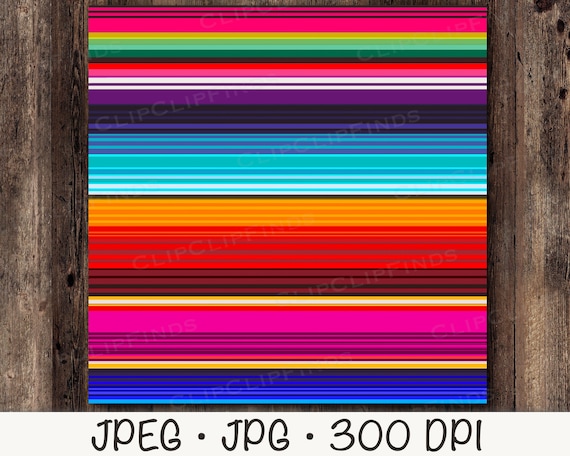The image in question is a vibrant and eye-catching digital graphic, set against a rustic, weathered dark brown wooden background that reveals its wood grain. Dominating the center of the image, slightly elevated with a drop shadow for added depth, is a nearly square rectangular banner. This central banner is filled with a series of horizontal lines, each a different and striking color, including various shades of blue, orange, yellow, red, green, turquoise, white, purple, magenta, black, and olive green, among others. The lines do not follow any discernible pattern and create a mesmerizing, colorful display.

At the bottom of this vividly striped banner, there's a small, funky Comic Sans-like font in black that reads "JPEG 300 DPI," clearly indicating details about the image format and resolution. This text sits within a white bar, further enhancing the graphic's distinctive look. The image overall has a stylish, somewhat retro aesthetic, reminiscent of visual patterns seen on late-night television sign-offs or old notebook designs. It could serve as a digital download, a product photo, or even as a striking wall decoration.